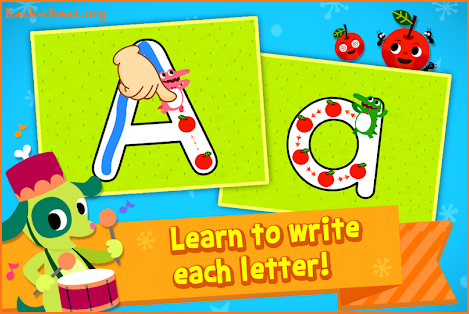The image appears to be a colorful, cartoonish educational graphic, likely sourced from or related to the website hackcheat.org, as indicated by the text in the upper left corner. The background is a vivid blue, and the main focus is on two large squares that resemble children's alphabet blocks.

The block on the left features a capital "A" in white, accompanied by a hand diagram illustrating how to write the letter. The block on the right displays a lowercase "a," alongside images of a red tomato, a green alligator, and possibly another small green creature. These images are designed to be visually engaging for children, likely to help them associate the lowercase "a" with words like "alligator" and "apple" (although the fruit depicted seems more like a tomato).

Above these blocks, there is text that reads "Learn to write each letter," reinforcing the educational purpose of the image. Additionally, two small, round-headed cartoon characters, resembling smiling tomatoes or apples, are positioned above the blocks. The entire graphic is brightly colored and designed in a fun, approachable style to appeal to young children learning the alphabet.